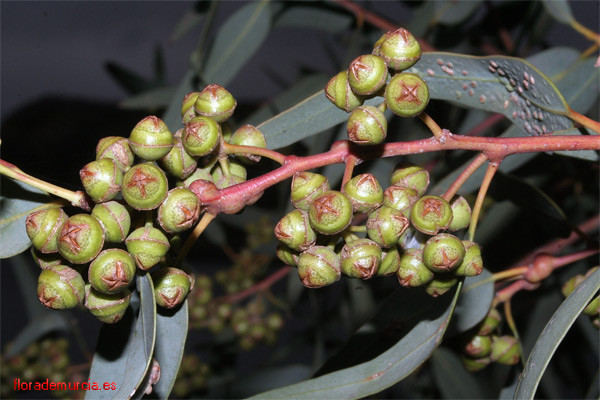The image captures a red tree branch adorned with clusters of unusual green acorn-like berries, each marked distinctly with a red X at the base. These berries, possibly nuts, are grouped in varying numbers: a cluster of six, a cluster of around 15, and a larger cluster of about 20. The branch, bearing the texture and appearance of acorns, is surrounded by muted green-gray leaves with faint red speckles, resembling eucalyptus. The background hints at more trees and a sparse arrangement of additional leaves. The photograph appears to be taken at night with the flash illuminating the scene, accentuating the glossy, almost plastic-like shine of the berries. At the bottom left corner of the photo, red text reads "flora demurcia.es," indicating a possible link to a floral arrangement website.